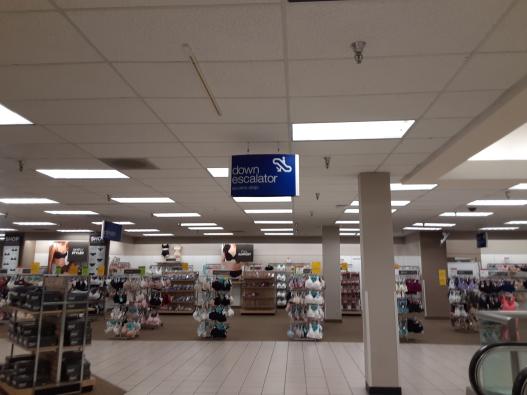The image captures the interior of a department store, revealing a wide-angle view that encompasses multiple sections. Dominating the ceiling is a blue sign that reads "Down Escalator," with the escalator itself partially visible in the bottom right-hand corner. The ceiling is a white drop style, equipped with numerous rectangular fluorescent lights and sprinkler nozzles, supported by large, nondescript square columns featuring dark-colored bases. The floor transitions from light gray ceramic tile in the main circulation area to brown carpeting in the sales sections. On the left side, gray shoeboxes are organized on shelves, and prominently to the back are racks adorned with women's lingerie, including bras. Enhancing the display, images of models wearing black bras decorate the left side of the picture. The store's overall layout and features evoke the feel of an old Sears, with its practical tile flooring and functional beam structures.